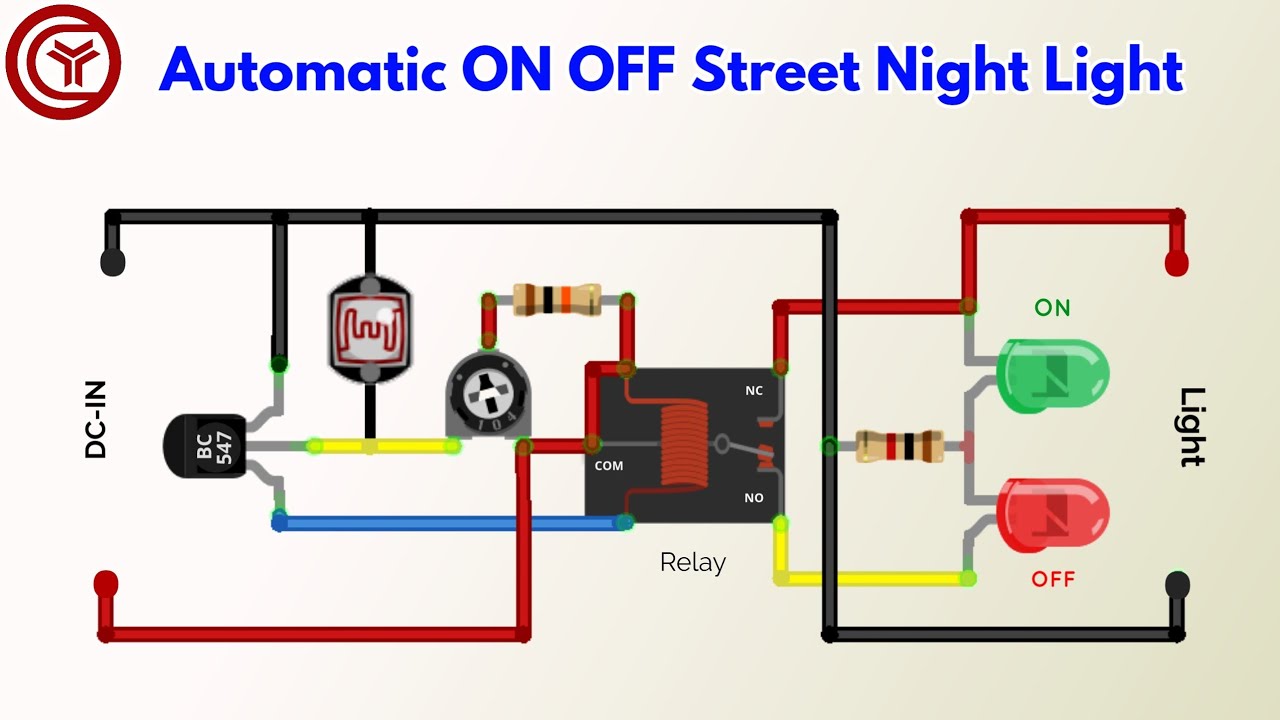This is a detailed 2D diagram illustrating the mechanics of an automatic on-off street nightlight. At the top of the diagram, the title "Automatic On and Off Street Nightlight" is displayed in blue, accompanied by a red logo in the top left corner. The left side of the diagram is labeled "DC In," where a black wire runs horizontally before curving around to connect with a relay in the middle. A parallel red wire also originates from "DC In," running and curving around, touching various components.

The relay, prominently positioned in the center, is marked with the label "relay" and includes a small switch. It features connections involving multiple wires: a red wire, a yellow wire which links to an on-off switch, a blue wire, and another yellow wire leading to a component labeled "BC 547."

On the right side of the diagram, there are two diodes, one red and one green. The green diode illuminates when the circuit is on, while the red diode lights up when the circuit is off. The colors used in the diagram—red, yellow, green, and blue—make it vibrant and easy to follow, providing a clear and informative visual explanation of how the automatic street light operates by transmitting signals to activate the lights depending on the conditions.